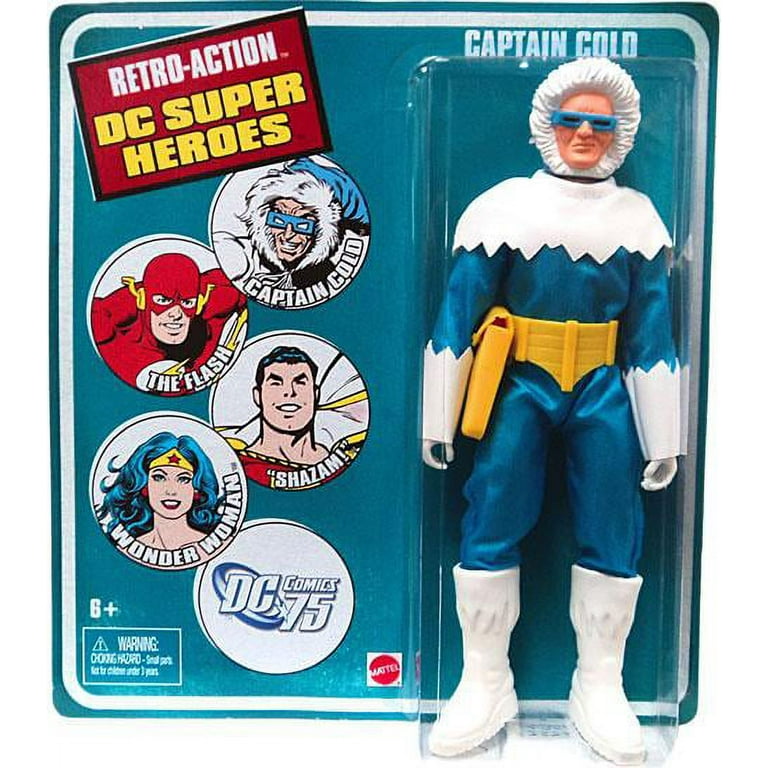This image features a vintage-style DC Superheroes action figure of Captain Cold, part of the DC Comics 75 series. The toy, produced by Mattel, bears the "Retro Action" label, suggesting it is either a recent release designed in the style of late 80s to early 90s toys or an actual vintage piece. Captain Cold is depicted in his signature cold suit: a blue outfit with white trim, large white boots, and a big yellow belt that includes a pouch. He also wears a hood and blue glasses, resembling 3D glasses, which emphasize his cold-themed persona. The packaging, simple and clear plastic, displays images of other action figures in the series, including Wonder Woman, Shazam, and The Flash. The bottom of the packaging includes a "DC Comics 75" bubble, an age recommendation of "6 and up," a Mattel logo, and a choking hazard warning.